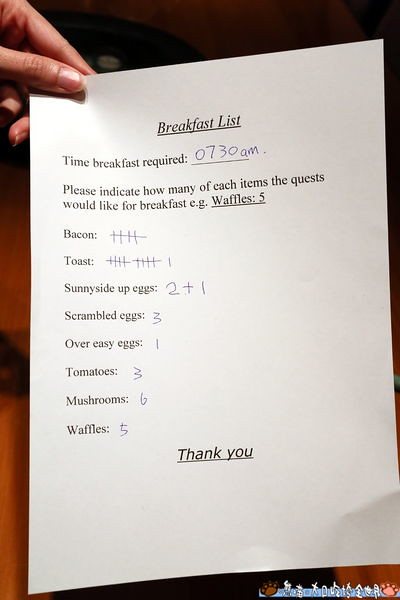The image showcases a white breakfast menu held by a woman's left hand, identifiable by her polished fingernails. The menu prominently displays the title "Breakfast List" at the top. Below that, the printed text reads, "Time breakfast required," with "0730 AM" handwritten alongside. Further down, the instructions ask guests to indicate the quantity of each breakfast item they desire, listing examples as follows: waffles 5, bacon 5, toast 11, sunny side up eggs 2 + 1, scrambled eggs 3, over easy eggs 1, tomatoes 3, mushrooms 6. The document concludes with a courteous "Thank you." At the lower right corner of the paper is a white and blue logo, which is somewhat indistinct. The overall setting suggests that this is a self-fill breakfast menu likely used in a hotel or convention setting.